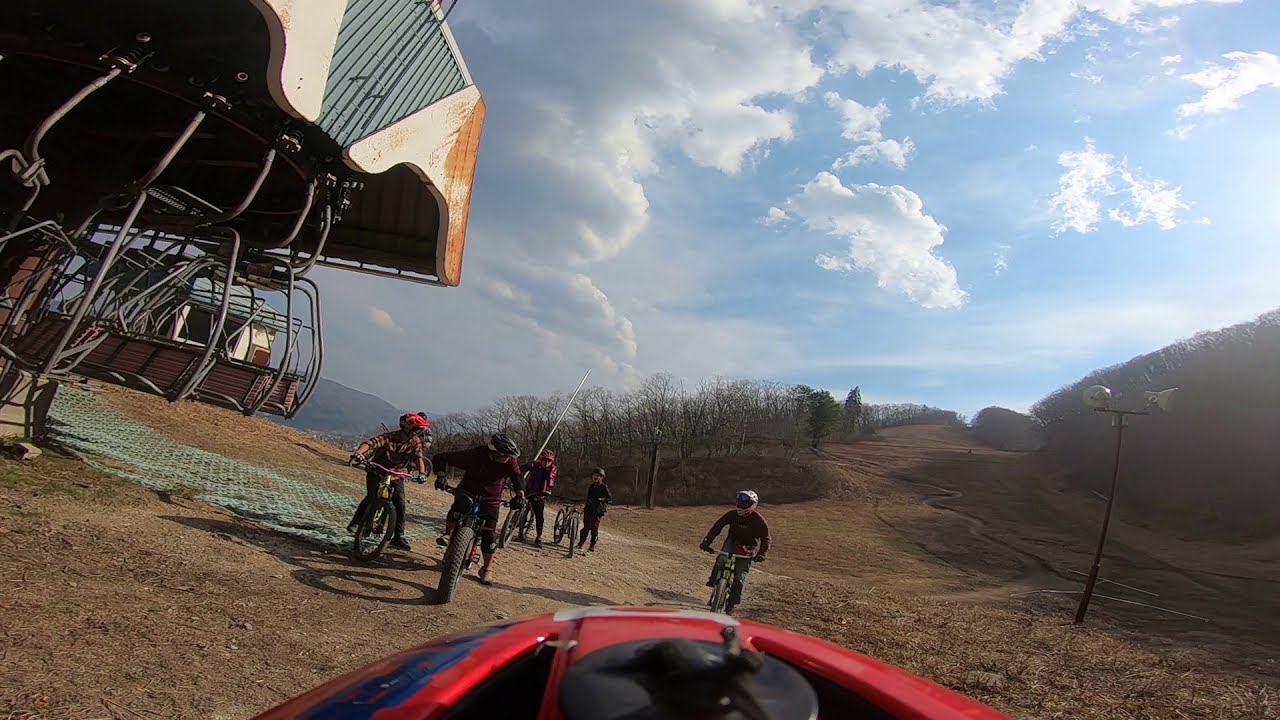The photo depicts a lively scene of six cyclists, likely comprised of kids and teenagers, gathered in an open, summer landscape that is clearly a ski area during its off-season. The trail appears to stretch out long in front of them, winding through a terrain mostly covered in dirt, with some patches of grass. The background is rich with trees, their branches bare, suggesting it might be a transitional season. 

The riders are positioned in the middle ground of the image; three of them are mounted on their bikes, ready to continue moving, while two stand beside their bikes, possibly taking a short break. To the left, the remnants of winter activities are evident, most notably a ski lift and some scattered equipment, possibly related to either skiing or biking. On the right, a wide, dirt hill ascends, emphasizing the higher elevation of the scene.

The sky is partly cloudy, providing a bright but not overly sunny day, ideal for such an outdoor adventure. The photograph is rich in earthy and natural tones—blues, whites, browns, greens, blacks, and reds—all contributing to the vividness of this active and engaging outdoor moment.